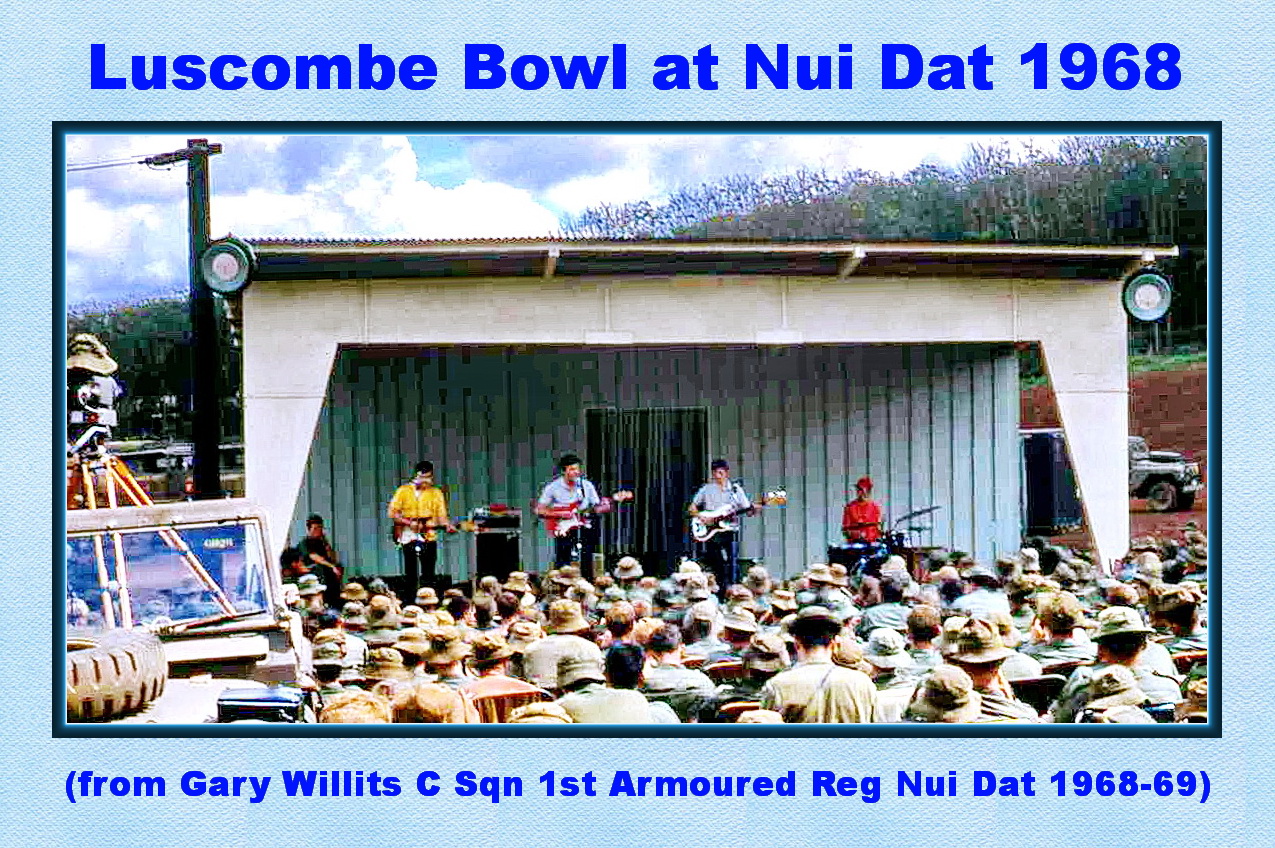The landscape image features a concert scene from 1968. At the top, the text "Les Combes Boule at Nui Dat 1968" is overlaid in bright blue, while the bottom reads "From Gary Willett, C, SQN, First Armored Reg, Nui Dat 1968-69." The center of the image is dominated by a photograph bordered in black. The concert is set on a small stage with a white overhang, a blue background, and siding. Four people perform on stage—three playing guitars and one on drums—with another person sitting in the corner, possibly watching. The audience, visible from behind, wears various shades of green fatigues and hats, seated in chairs in the open air. The background shows trees, dirt, sky, and poles, with the front of a vehicle and a spare tire visible in the lower left-hand corner.